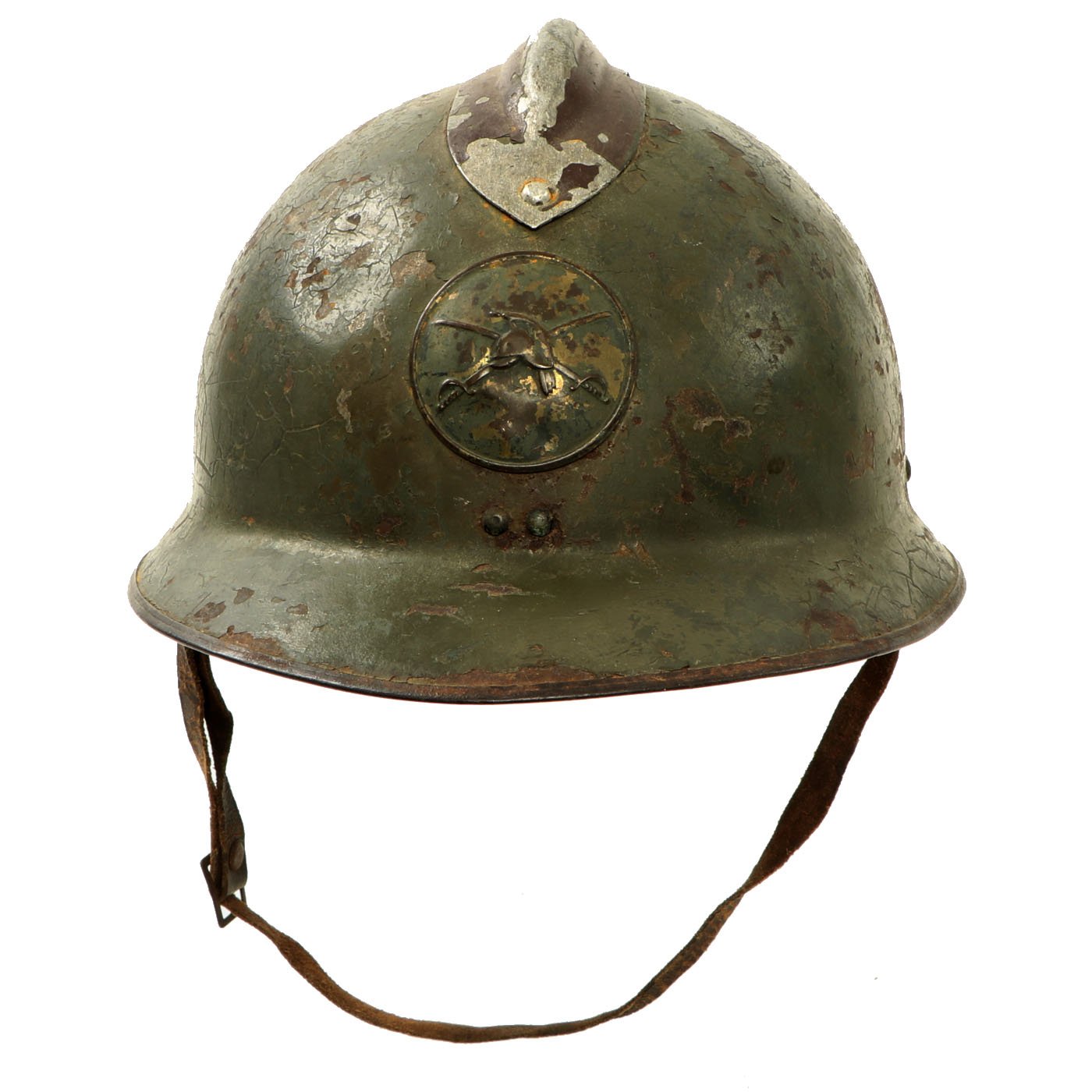This image features a historical military helmet, likely from one of the early World Wars, distinguished by its age and wear. Constructed from green-tinted iron, the helmet exhibits extensive rust, chipped edges, and various imprints suggestive of battlefield use. The front center of the helmet is adorned with a circular emblem depicting two crossed swords behind a smaller helmet, characteristic of European design. A leather chin strap hangs from the bottom rim, accentuating its authenticity. The top of the helmet has a distinct addition: a silver-colored metal fin resembling a mohawk. This finely detailed artifact, with its textured damage and debris, appears well-suited for display in a museum, providing a vivid glimpse into military history. The photo quality is clear with ample lighting, allowing all these features to be readily observed.